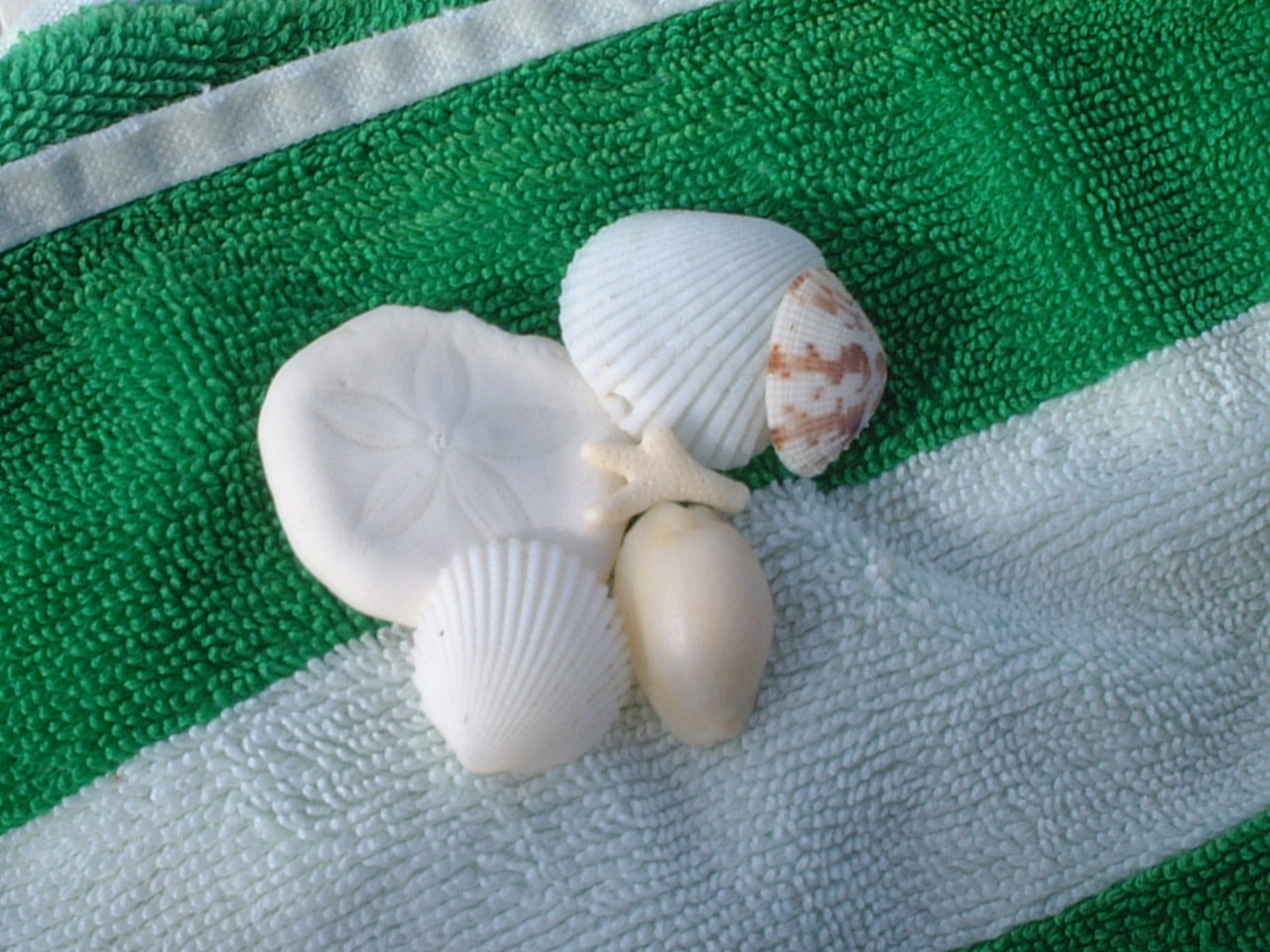This close-up photograph captures six seashells artfully arranged on a crisp, green towel with white stripes and a white border, seated atop a gray or white surface. In the top left corner lies a delicate sand dollar, accompanied to its right by a white shell. Further to the right is another white shell with distinctive brown markings. Below these lies an additional white shell paired with a cream-colored shell. Among the group are two classic clamshell varieties, reminiscent of those from famous paintings, featuring ridges and a pristine white color. Additionally, there is a small, spiral-shaped shell and a tiny piece of coral. Grouped together without any sand, the cleaned shells suggest they were carefully collected from the beach.